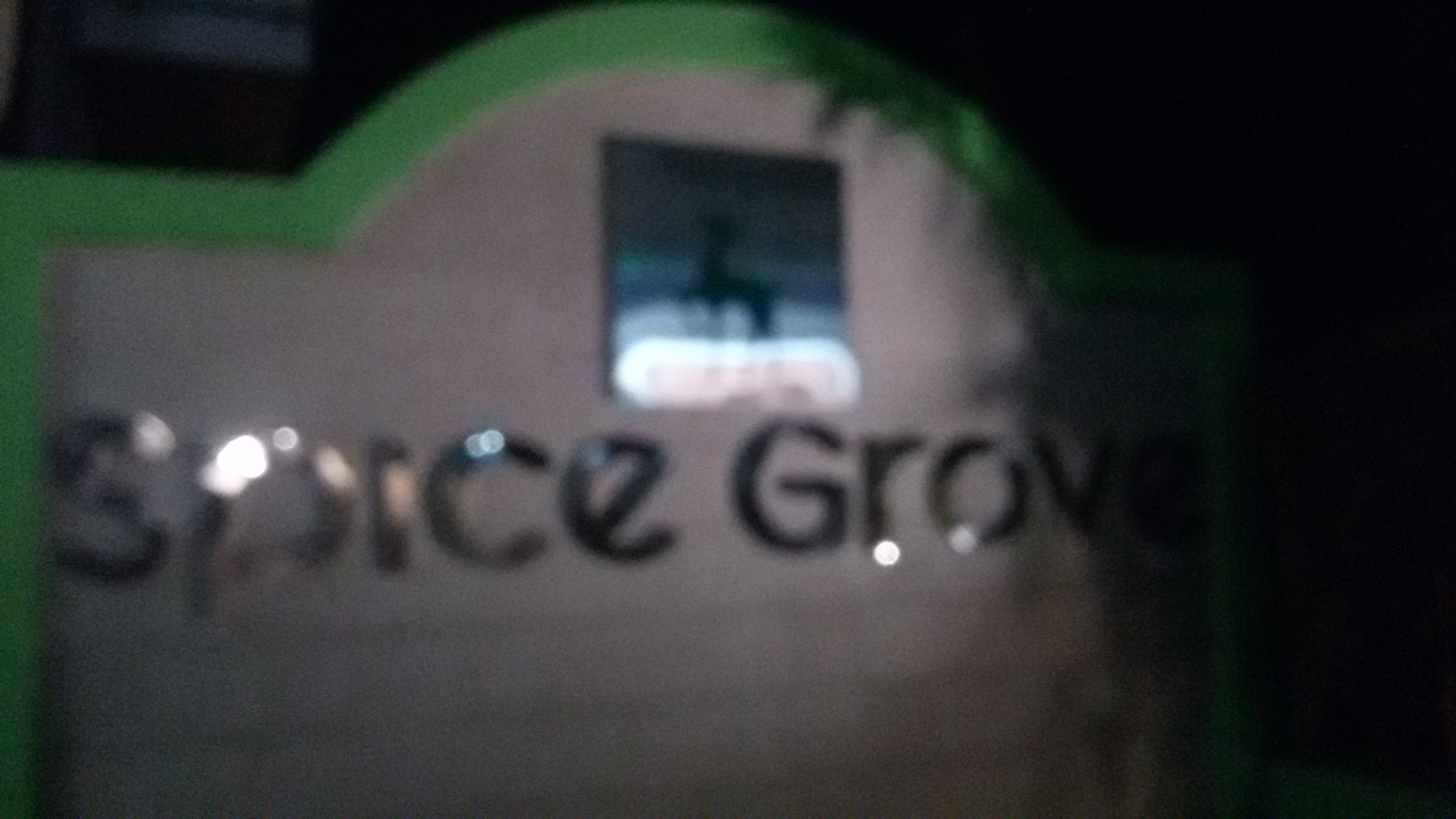A night-time outdoor photograph, despite its blurry and low-quality nature, captures a large street sign made from white brick with a yellowish stone border. The sign, reminiscent of those typically found at the entrance of malls or strip malls, is rectangular with a distinctive circular protrusion on top. Beneath the circular section, there is an image or poster featuring a silhouette of a deer in a pirouette stance. Below this artistic depiction, the sign displays bold black plastic letters spelling out "Spice Grove."